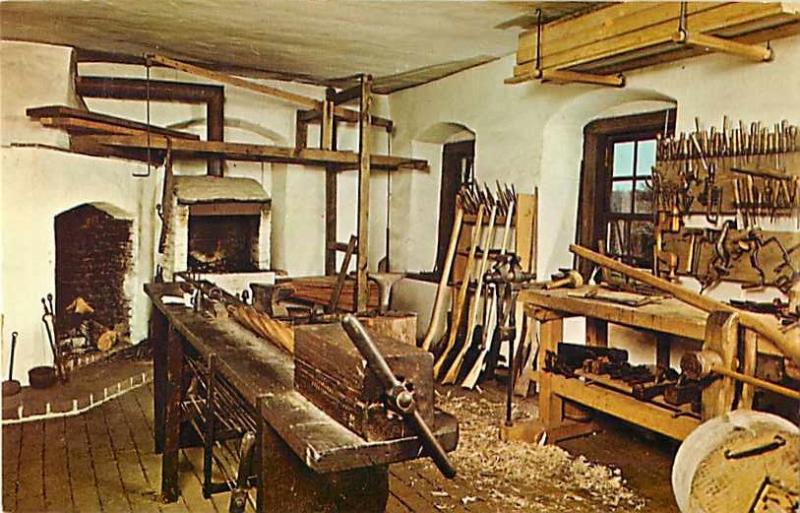The image captures a detailed view of an old, active woodworking shop, probably dating back to the 1960s or 70s, housed inside a cabin-like structure. The workshop is bustling with activity, evident from the sawdust scattered across the wooden, possibly tiled, floors. The room has a distinct adobo style with rounded doorways and window frames, featuring predominantly whitewashed, concrete-like walls accented with warm, orangey tones, contributing to an aged, nostalgic aesthetic.

The shop is replete with woodworking tools, including a workbench cluttered with chisels and various shaping instruments. A wooden vise with a metal rod is visible, used for securing wood pieces for detailed work. Suspended from the upper shelves are neatly strapped wood planks, ready for future projects. A lathe with a spinning piece of wood, potentially an oar or rifle stock, symbolizes the ongoing work.

Two brick fireplaces, integral to the room's heating and woodcraft technique, are strategically positioned—one on the lower left side and another in the background. These fireplaces indicate the use of traditional methods, such as burning designs into the wood. Long hunter rifles are propped against the wall, suggesting the shop might also cater to hunting enthusiasts or produce custom firearms.

The cabin’s motif, a blend of white and natural brown hues, along with the vintage woodworking equipment and tools, reflects an era gone by, painting a vivid picture of an industrious yet warm and rustic workshop environment.